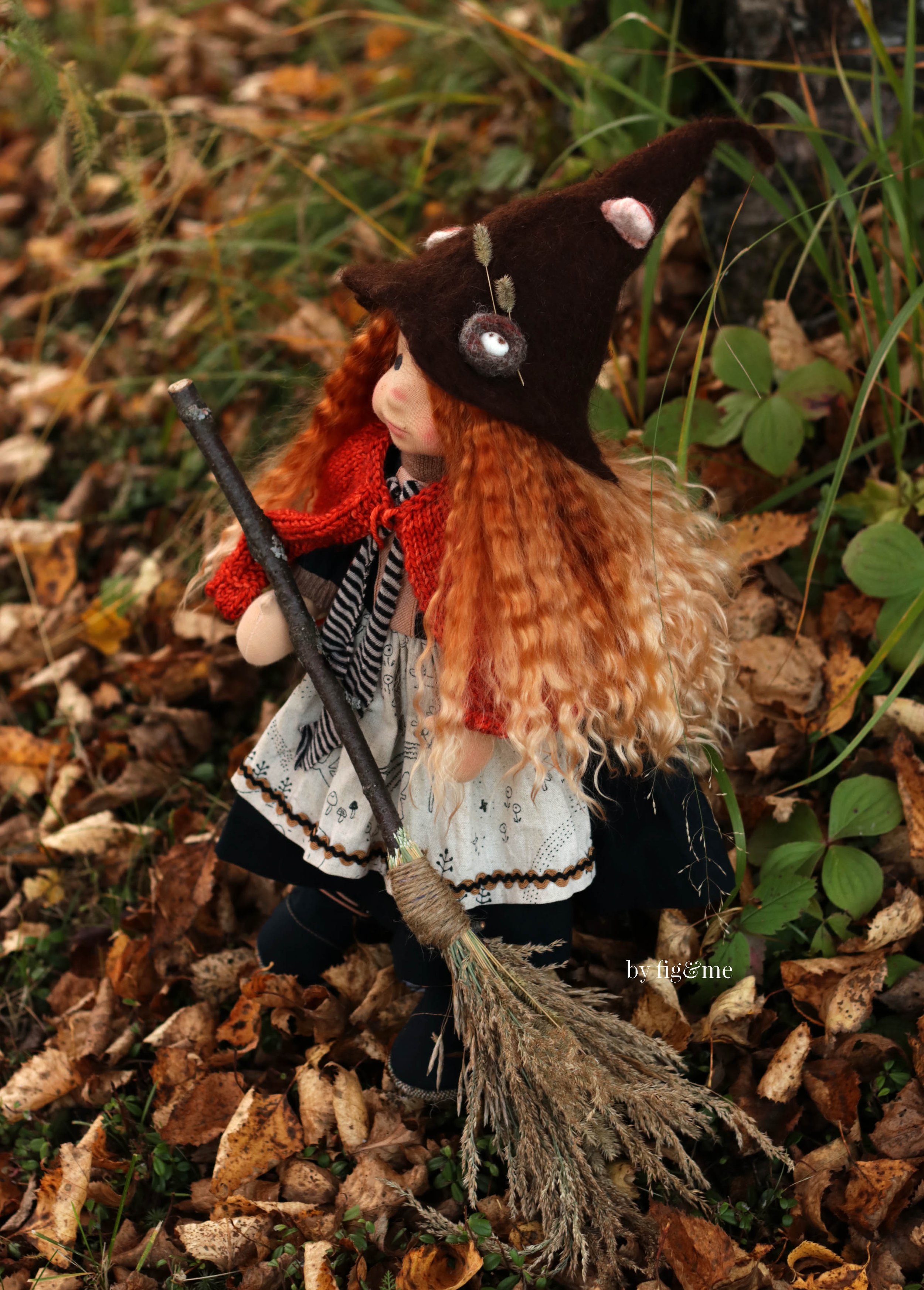This detailed, portrait-orientation color photograph showcases a whimsical miniature witch figurine named Glinda, crafted or manufactured by the brand "By Fig and Me," as indicated by the small white logo in the bottom right corner. The central subject of the image is a small doll dressed as a witch, positioned on a grassy ground outdoors, surrounded by brown leaves and green plants in the background. She wears a pointed black hat adorned with stitched objects, a black and white dress complemented by a white apron, and a red scarf around her neck. Her long, curly reddish-blonde hair cascades down her sides. In her right hand, she holds a broom composed of a black handle and a natural brown sweeper part, tied off with a rope, adding to the natural fiber art aesthetic. The composition, rich in realistic photographic representationalism, places the doll centrally, creating an enchanting scene reminiscent of a garden gnome in a yard, yet distinctly characterized by her witch-like appearance and attire.